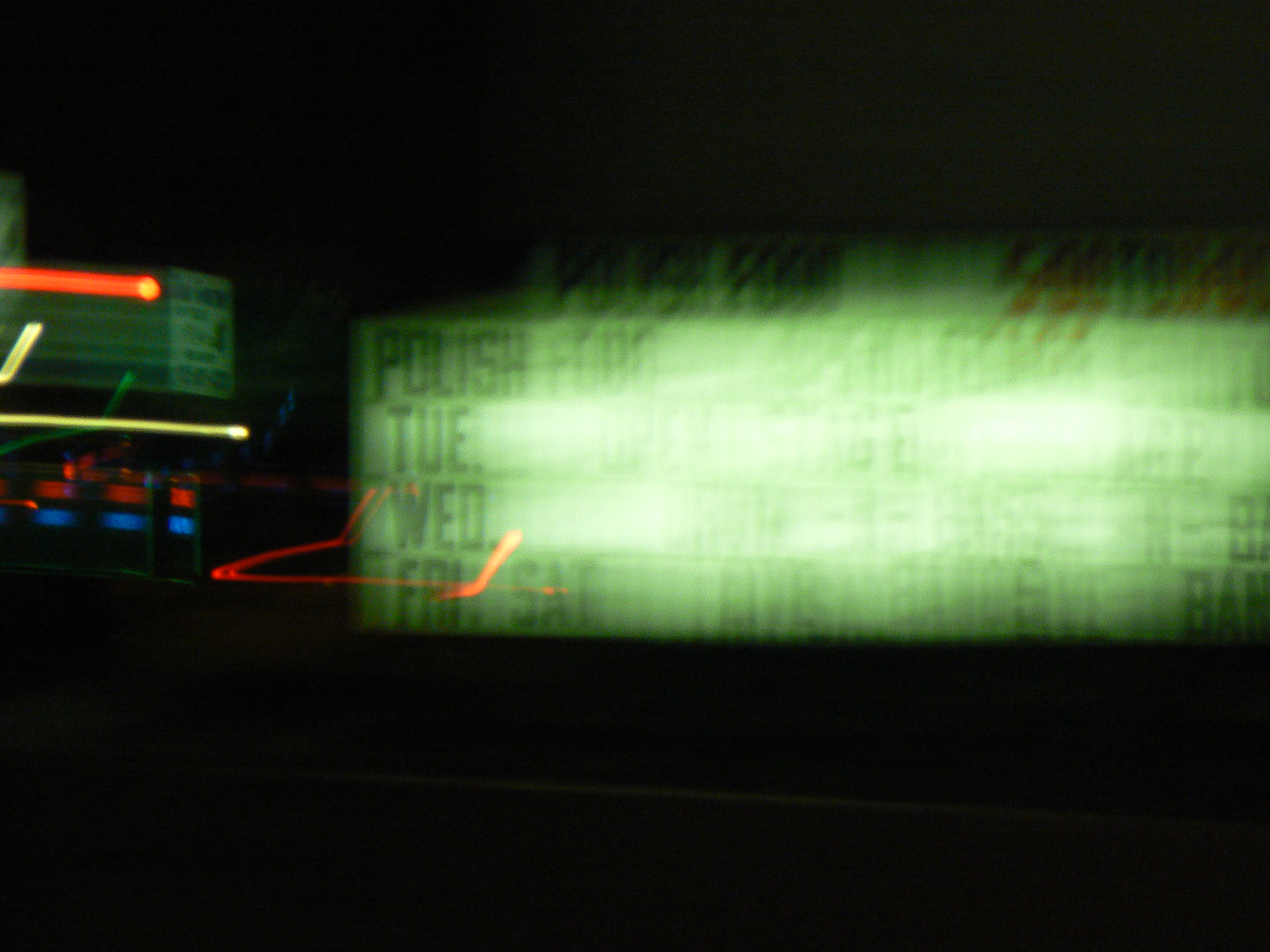The photograph appears to have been taken at night from a moving vehicle, which results in a blurred effect and glare from various lights. On the left side of the image, there is a structure with a large neon blur, possibly showcasing a window with a red and blue neon sign. Dominating the center and right side of the picture is a rectangular theater-style signboard, where letters are individually positioned to form words. The sign reads "Polish Food" on the top line, followed by "Tuesday" on the second line, "Wednesday" on the third line, and "Friday and Saturday" on the fourth line. The text beyond that point is obscured by a significant glare, likely from the lights on the rest of the signboard.